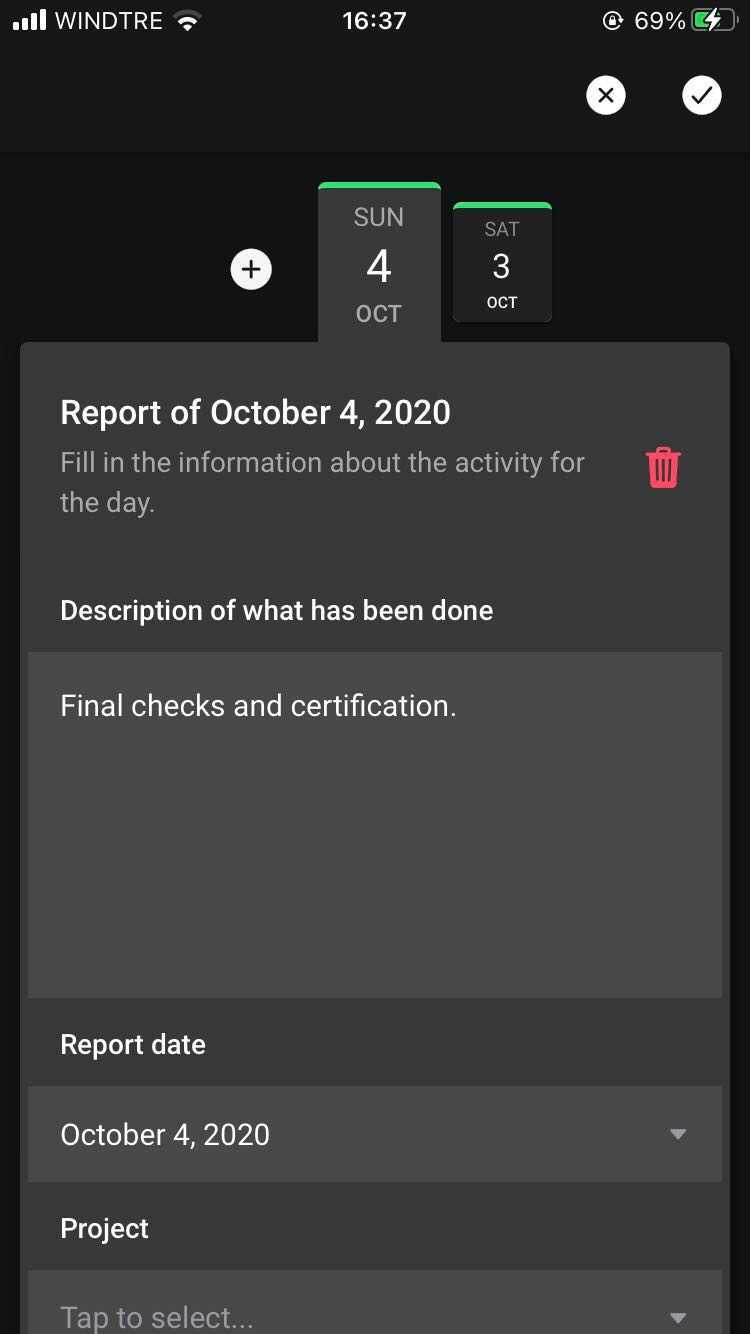The screen displays a detailed report interface with a predominantly dark color theme. In the top left corner, the status bar shows full signal strength and battery at 69%, alongside indicators "WIIN TRE" and 1637. Icon buttons for actions include a "Y" in circles for options, an "X" in a checkmark for confirmation tasks, and a red trash can for deletion. The interface lists entries for Sunday, October 4th, and Saturday, October 3rd, with the main report date set to October 4th, 2020. 

A drop-down menu labeled "project" prompts the user to select a task. The instructions read: "Fill in the information about the city for the day." Visible elements include descriptions of completed tasks, encompassing final checks and certifications. The visual setup centers around the efficient logging and reporting of data with clear action items indicated by easily recognizable icons.